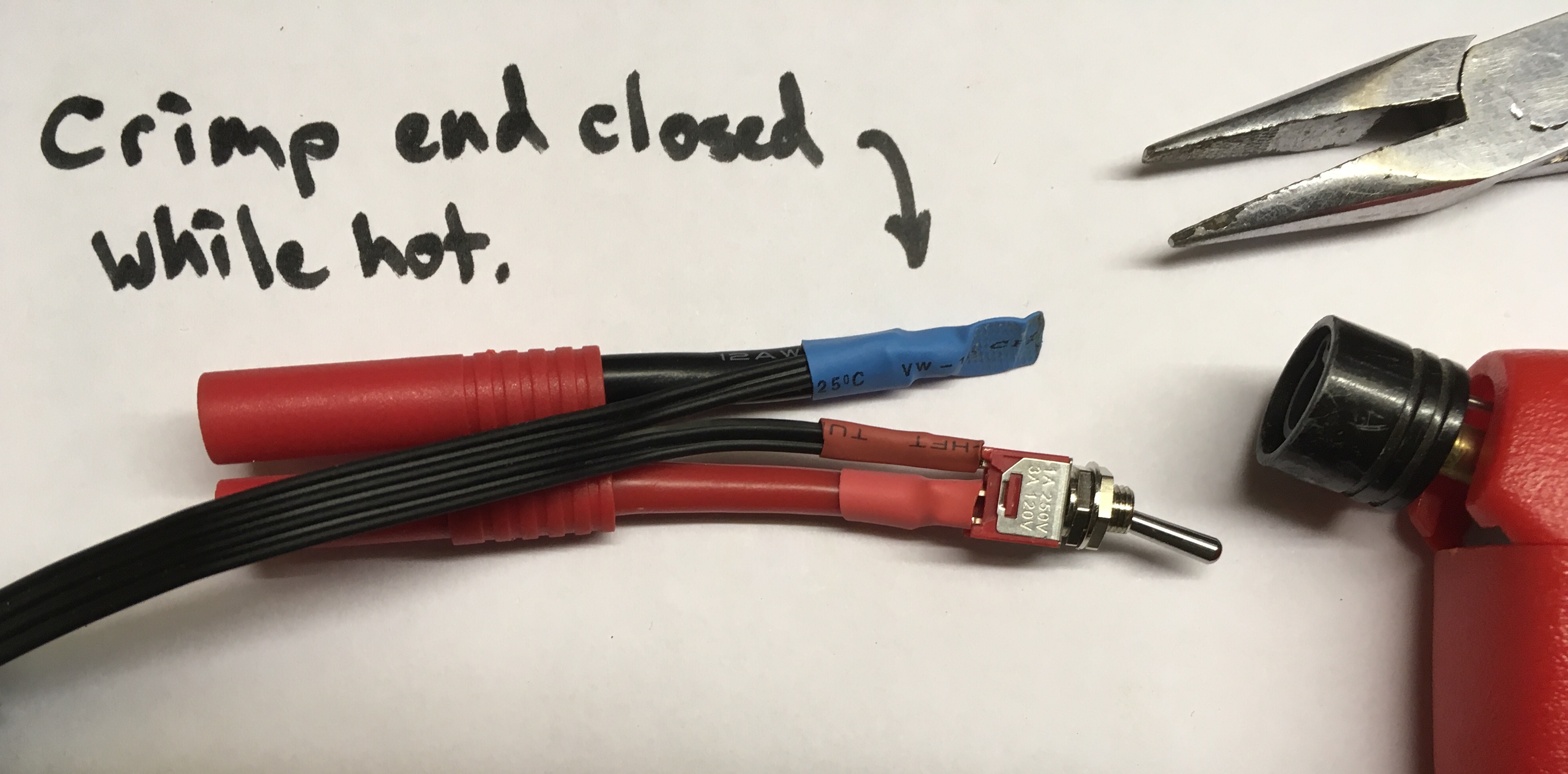This image features a plain white background with handwritten instructions in black Sharpie that read, "crimp and close while hot," accompanied by an arrow pointing towards a blue-tipped wire. The image displays a pair of needle-nose pliers in the upper right corner and a small blowtorch positioned below. There are two black wires: one tipped with blue tape, and the other tipped with red tape. Each wire has a large red cap with a divoted end. The red-tipped wire is additionally fitted with a metal switch, a bolt, and a metal piece connecting it to the switch. The overall setting appears to be an organized workspace.